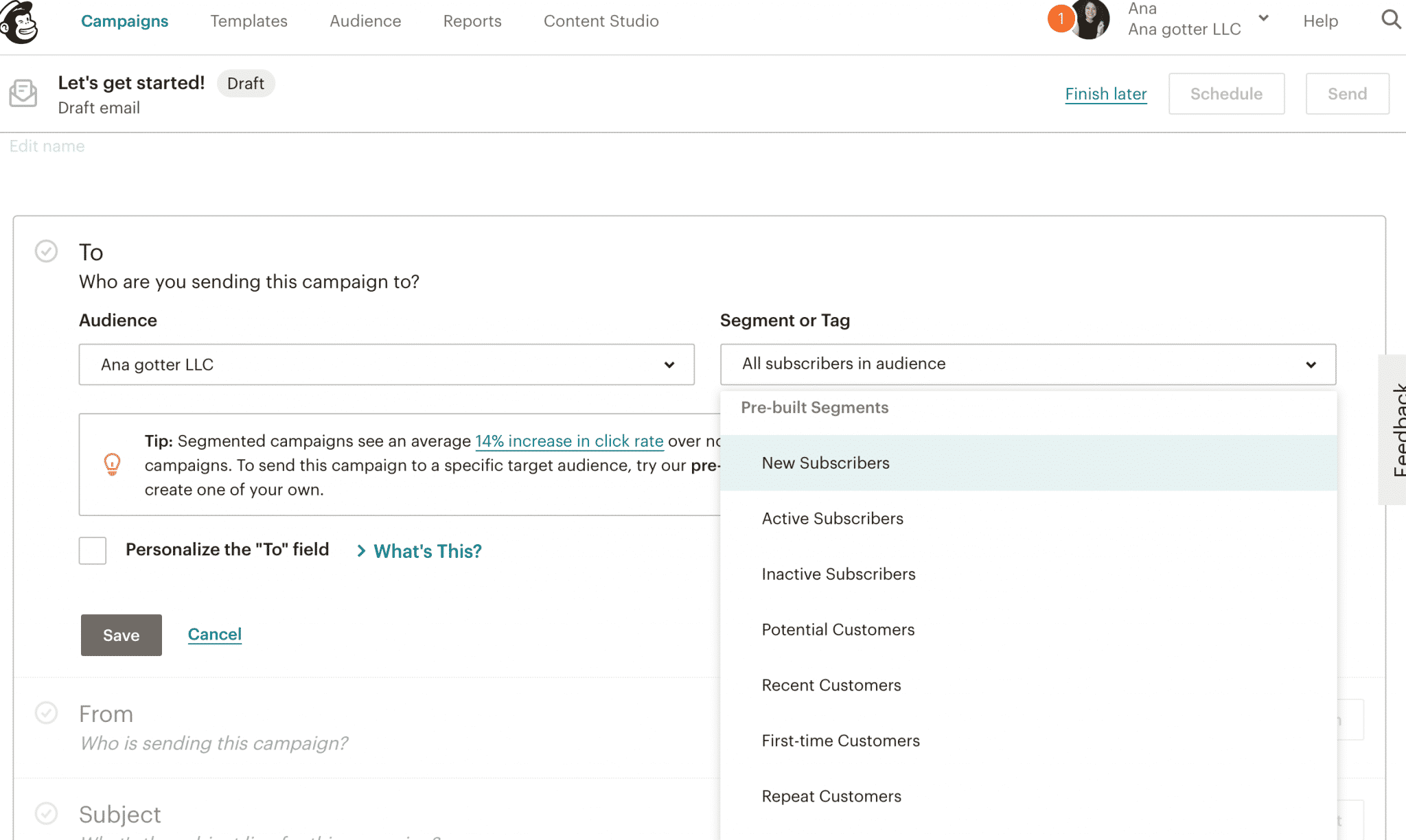**Screenshot of Email Campaign Dashboard in Marketing Software**

The screenshot features an interface from a marketing software platform, with various elements displayed. In the top section, there is a profile icon with the picture of a woman, accompanied by an orange notification circle with the number one. The profile name is "Anna."

On the left sidebar, several menu options are listed in blue, including:
- Campaigns
- Templates
- Audience
- Reports
- Content Studio

Just below the profile and menu options, there's a search bar with a magnifying glass icon and a help option.

Central to the image is a section titled "Let's Get Started," featuring a gray oval button marked "Draft." An email draft, indicated by the text "Draft Email - Finish Later," is presented in a blue rectangle. This section also includes buttons labeled "Scheduled," "Send," "Edit Name."

The next section prompts the user with the question, "Who are you sending this campaign to?" Below this question, there's an audience selector within a rectangle, listing "Anna Gotter LLC." Next to it is a tip icon.

Within this section, a checkbox allows users to "Personalize the 'To' field," with the 'To' word enclosed in quotation marks. A small "What's This?" link in blue offers additional information. Buttons for "Save" (gray) and "Cancel" (blue) are positioned at the bottom.

Further down, details for "From," "Circle," "Subject," and "Segment or Tag" are displayed. The "Audience" dropdown menu shows options with pre-built segments highlighted in blue, listing:
- New Subscribers
- Active Subscribers
- Inactive Subscribers

Overall, the image depicts a comprehensive overview of creating and managing an email campaign within the marketing software.